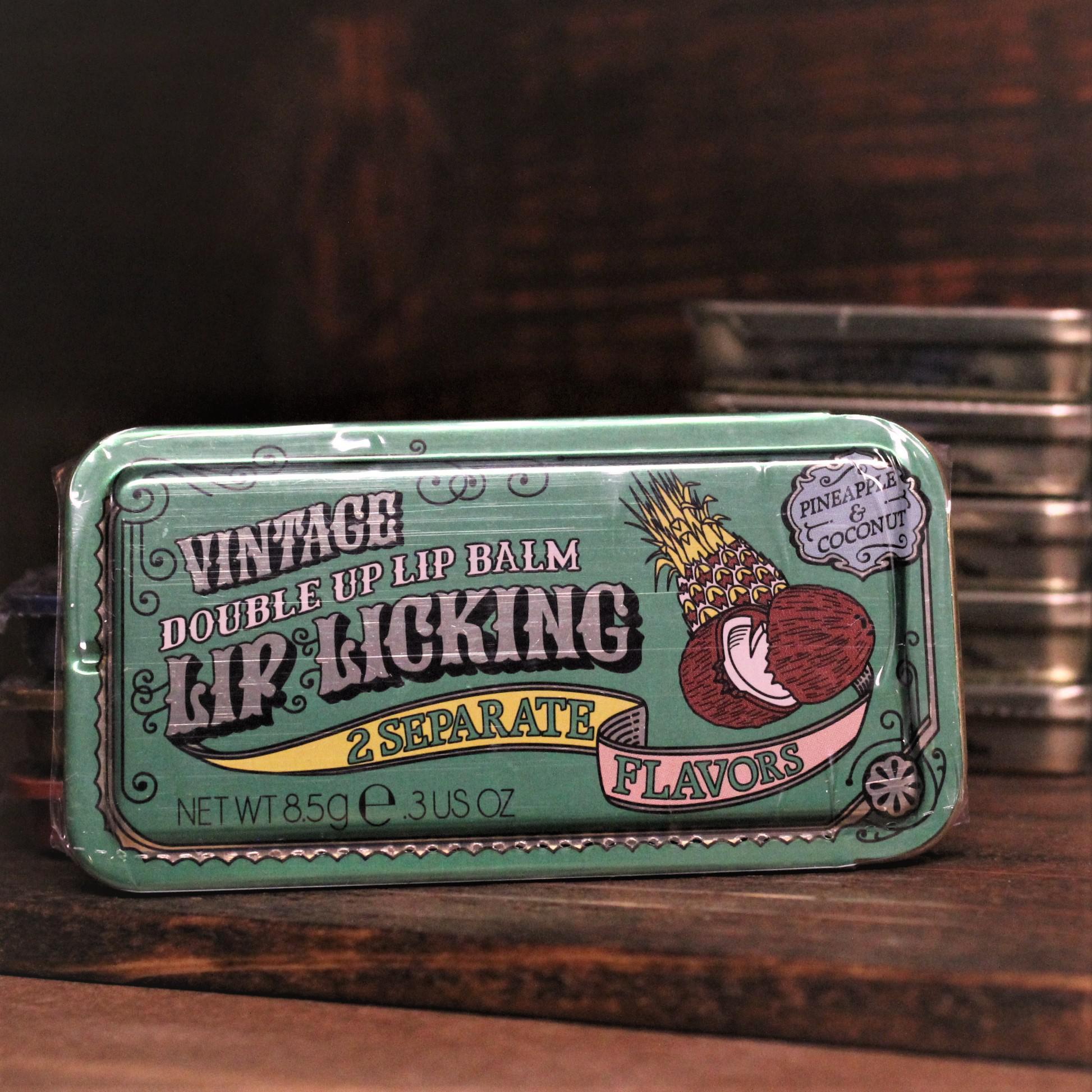This photograph, likely taken indoors, features a close-up of a unique rectangular metal tin, reminiscent of a sardine can, which contains a lip balm. The central tin, which is still covered in plastic, is teal-colored and prominently displays numerous detailed designs and texts. At the top, “Vintage” and "Lip Licking" are inscribed in a hand-drawn style with deep shadows and silver coloring. Below it, “Double Up Lip Balm” is written in white with a black outline. A banner in the middle of the tin states “Two Separate Flavors” with a yellow background behind "Two Separate" and a pink background above "Flavors." In the upper right corner, an ornate circle encloses the words "Pineapple and Coconut" in black font, accompanied by hand-drawn images of a split coconut and a pineapple. The net weight, 8.5 grams or 3 US ounces, is noted at the bottom left. Behind this highlighted tin, five more similar tins are stacked, although out of focus, on a dark, natural wood table, matching the dark wooden backdrop.